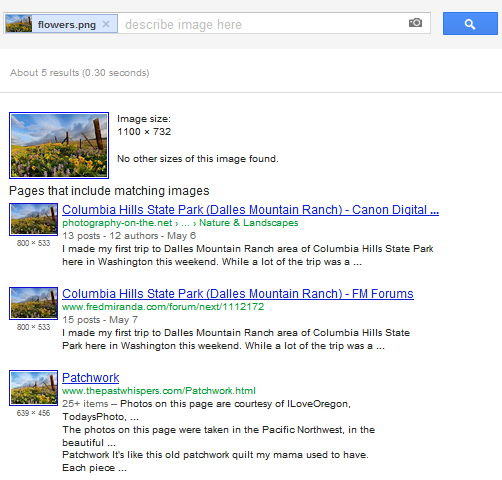Screenshot of a vintage-styled search engine, resembling an old version of Google. At the top, a search bar displays the query "flowers.png," with a note beneath indicating "about 5 results (0.30 seconds)." 

The first search result is an image with dimensions of 1100 x 732 pixels and a note: "No other sizes of this image found." Below the image, there are several matching pages listed:
- "Columbia Hills State Park, Dales Mountain Ranch"
- "Canon Digital Photography on the Net, Nature and Landscapes," featuring "13 posts by 12 authors, May 6," and a snippet stating: "I made my first trip to Dales Mountain Ranch area of Columbia Hills State Park here in Washington this weekend while a lot of the trip was a..."
- "Columbia Hills State Park, Dales Mountain Ranch," from "FM forums (www.fredmiranda.com/forum/next/1112172)," with "15 posts, May 7," accompanied by the same snippet as above.

The last search result is titled "Patchwork" from "www.thepastwhispers.com/patchwork.html."